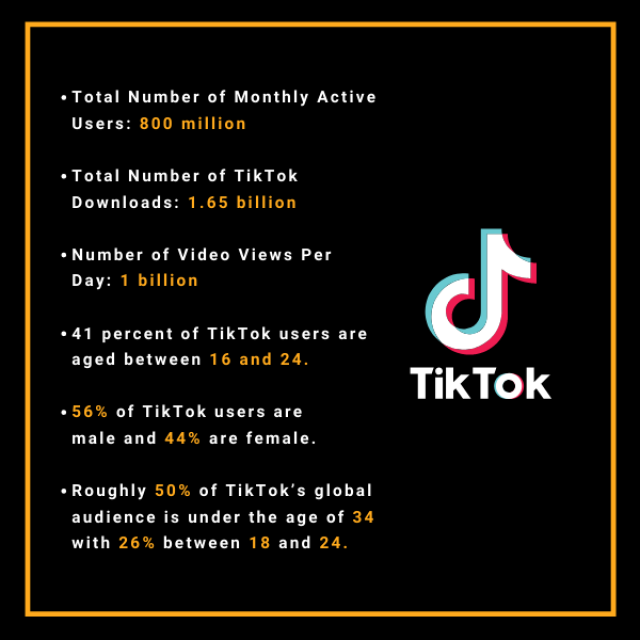**Infographic Data on TikTok Usage**

This infographic, set against a black background with a yellow-bordered frame, presents key statistics about TikTok's user base and engagement. On the right side, the TikTok logo - resembling a musical note shaped like a 'T' - is prominently displayed above the large, white-font text "TikTok." 

The left side features a detailed bullet list in white font, with critical data points highlighted in yellow:
 
- **Total number of monthly active users:** 800 million
- **Total number of TikTok downloads:** 1.65 billion
- **Number of video views per day:** 1 billion
- **Percentage of TikTok users aged between 16 and 24:** 41%
- **Gender distribution:** 56% of TikTok users are male, and 44% are female
- **Age demographics:** Approximately 50% of TikTok's global audience is under the age of 34, with 26% aged between 18 and 24

This combination of figures illustrates the widespread and diverse engagement with the TikTok platform globally.